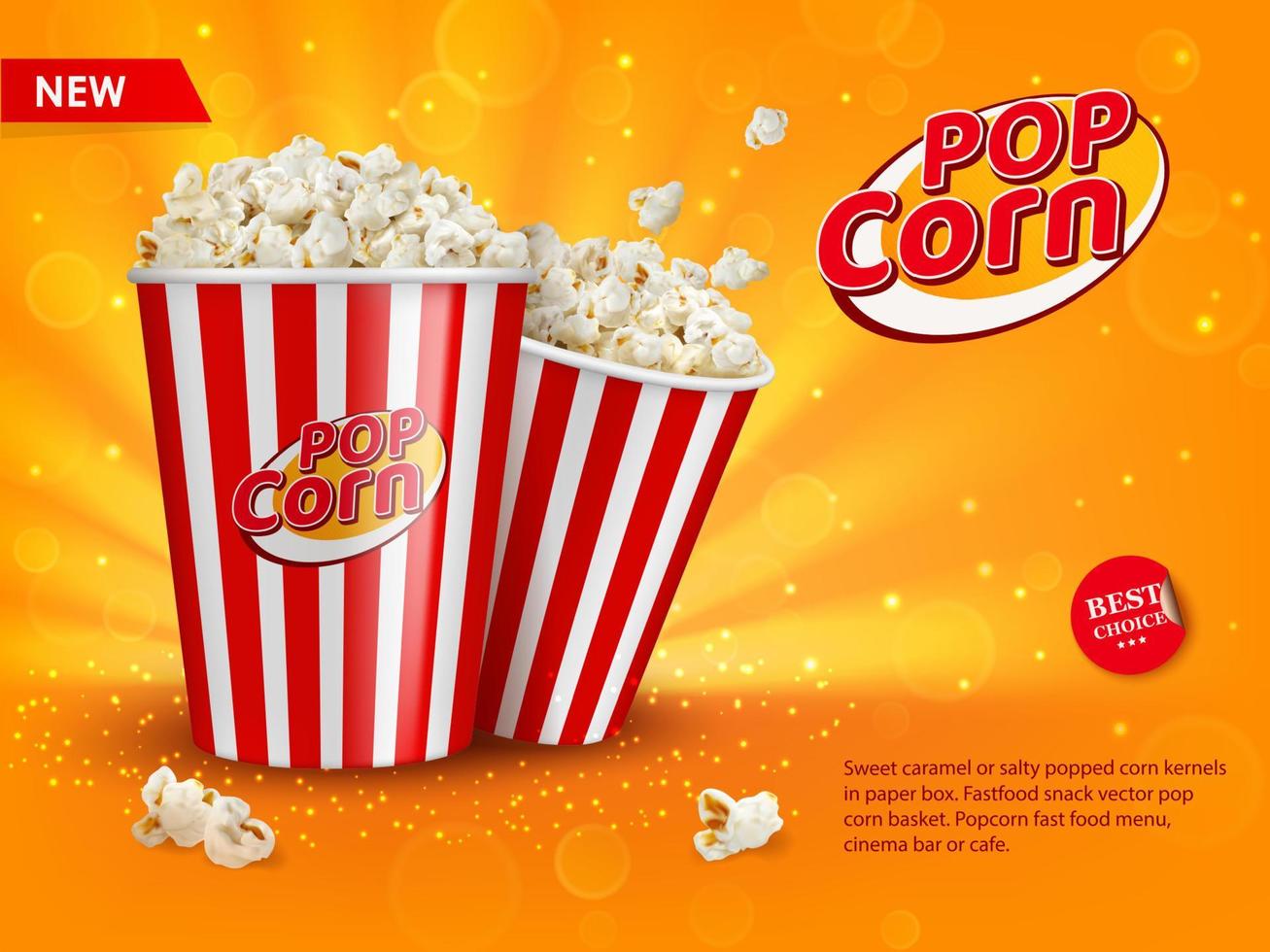The poster advertises popcorn, set against a vivid orange background with accents of red. Prominently featured are two cylindrical bowls brimming with plain popcorn, styled with classic red and white vertical stripes reminiscent of movie theater popcorn containers. The popcorn overflows, with a few kernels shooting out and some scattered at the base. In the top right corner, a popcorn logo is displayed, while another circular logo with a white border and the word "popcorn" in red appears on the side of the bowls, both suggesting branding for generic popcorn. The bottom right corner of the poster includes text offering "sweet caramel or salty popped corn kernels," indicating the flavor options. Nearby, a sticker reads "best choice," adding a seal of approval to the advertisement. White sparkles dotting the image lend a festive, glittery feel, enhancing the appeal of this tempting fast food snack suitable for a cinema bar or cafe menu.